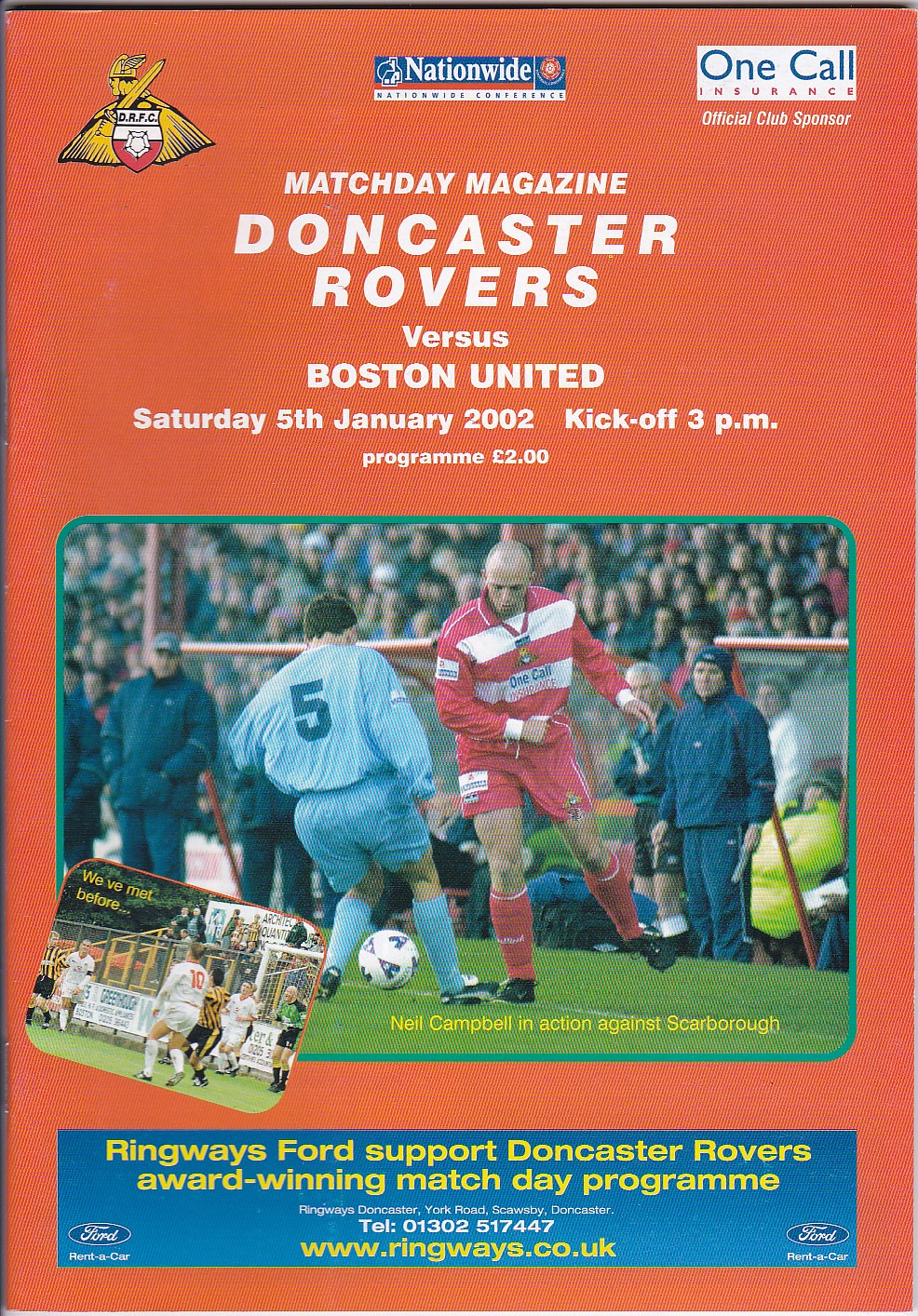Cover page of a vintage sports magazine, primarily orange in color, titled "Match Day Magazine." The upper third features the emblem of Doncaster Rovers Football Club (DRFC): a Viking character with a helmet and sword, looking from right to left, atop a gold shield. Adjacent to this emblem is the Nationwide Conference name and the logo of One Call Insurance, the official club sponsor. The main headline reads in white print: "Doncaster Rovers vs. Boston United, Saturday, 5th January 2002, Kickoff 3 p.m. Program £2."

A prominent, vivid photograph dominates the middle third: showcasing a tense moment from a soccer match. In the scene, a player in a red and white striped shirt, red shorts, red socks, and black shoes blocks a soccer shot from a blue-clad player, bearing the number 5. This action shot captures the intense rivalry and passion of the game, set against a backdrop of spectators and coaches attentively watching from the sidelines. Near this image, a smaller caption reads: "Neil Campbell in action against Scarborough."

The bottom third of the cover features a blue horizontal strip with a Ford commercial: "Ringways Ford support Doncaster Rovers' award-winning match day program." It includes the Ford logo, a telephone number "01302 517447," and the website "www.ringways.co.uk.” In this section, smaller imagery of another football match is also depicted, showing players in contrasting kits of red, black, and yellow stripes against those in all white, positioned in dynamic stances around the football field, with a visible goalkeeper in green near the goalpost. The words "We've Met Before" hovers over this smaller picture, providing historical context for the game.